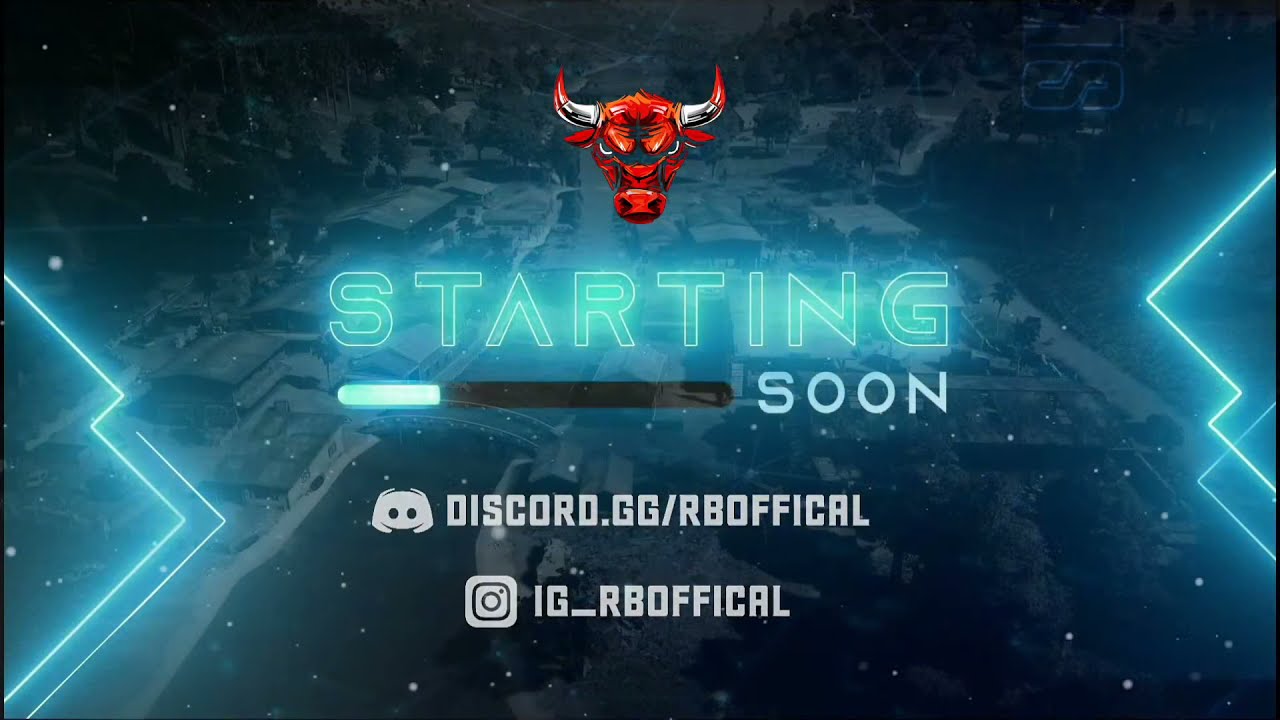The image appears to be a screenshot from either a YouTube video or a video game page on Discord. The background features a faded overhead image of a town with numerous small houses and trees, all tinted various shades of blue due to a blue overlay. On the left and right sides of the image, there are jagged neon blue lines that resemble mountain peaks or lightning, lending a Tron-like aesthetic.

In the center top of the image, there is a prominent red bull's head with silver horns that have red tips. Beneath the bull's head, in large electric blue outlined letters, is the word "starting," and adjacent to that in light blue font is the word "soon." A glowing blue progress bar, partially filled and inching towards completion, spans horizontally below the text, signifying that something is about to begin.

Towards the bottom of the image, in white font, are the Discord and Instagram details: "discord.gg/RBofficial" and "IG_RBofficial," indicating the social media connections related to the content.